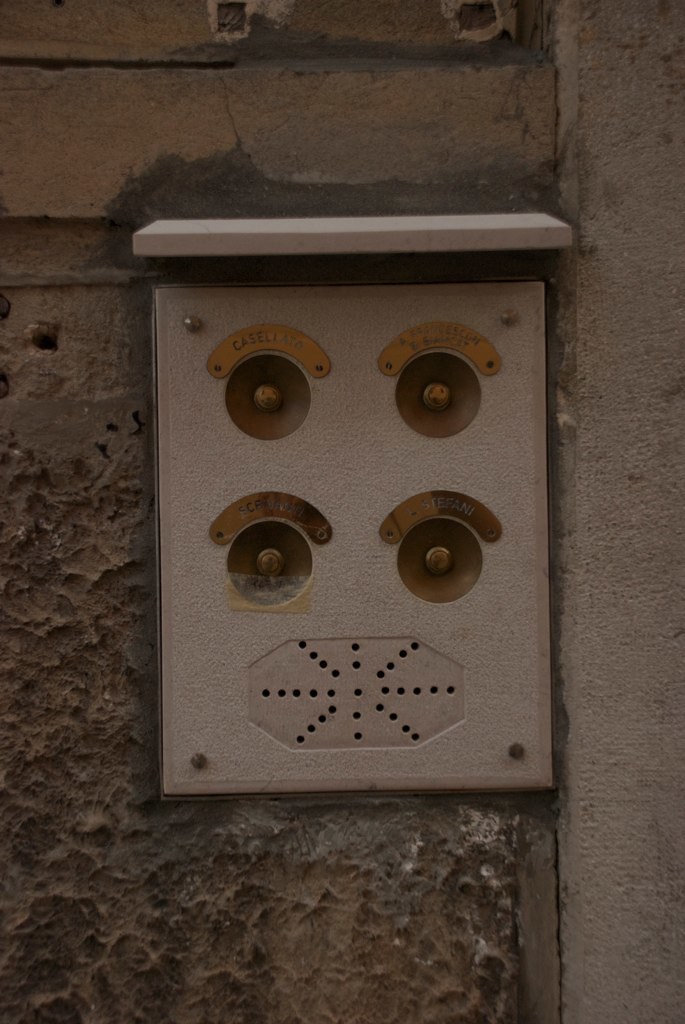The photo depicts an outdoor scene featuring a wall-mounted intercom system on the outer wall of a building. The structure is composed of a gray stone wall that displays significant wear, including various cracks and indentations, typical of a well-aged facade. On top of this deteriorated stone is a mix of materials, possibly bricks and a dark stony facade, adding to the texture and complexity of the image. 

At the center of the photograph is a rectangular, light white stone intercom unit. Above this unit, there is a small white stone ledge or awning extending from the main wall, likely serving to protect the intercom from rain. The device itself features an intricate design: at the bottom is an octagonal speaker with numerous small black holes arranged in diagonal and vertical patterns, resembling a stylized sun or lines on a basketball.

Above the speaker are four golden circular buttons, which are used to buzz inhabitants of the building. These buttons are accompanied by golden semi-circular nameplates with inscriptions, although they are somewhat difficult to decipher due to the image's darkness and wear on the intercom. Names such as "Caselato" and "Stefani" are faintly visible. The four buttons are surrounded by a faded central gold circular indentation, functioning as the buzzing mechanism.

The overall scene not only highlights the detailed texture and aging of the building materials but also captures the functional and aesthetic design of the intercom system, offering a glimpse into the building's entryway and resident communication system.